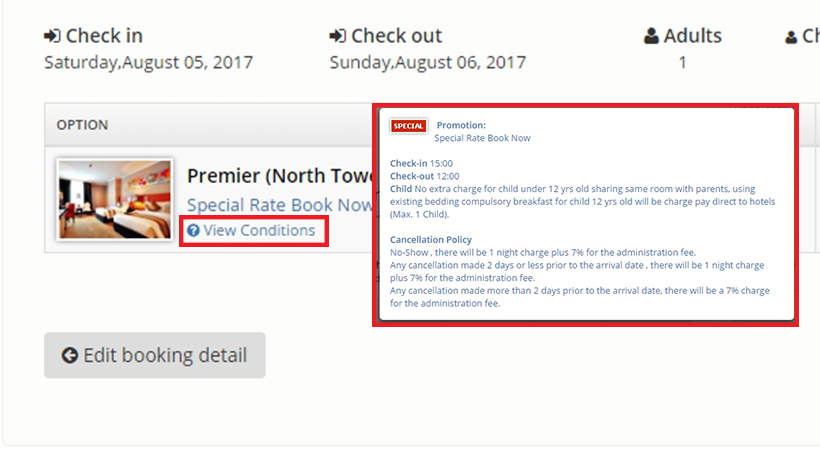The image is a promotional banner for a hotel booking website. The main component is a light grayish-pink box, prominently featuring key booking details. 

At the top, the header displays "Check-in" in bold black letters with a right-pointing arrow, followed by the date "Saturday, August 5th, 2017." Below, "Check-out" is shown in the same bold black font, accompanied by a right-pointing arrow and the date "Sunday, August 6th, 2017."

A section labeled "Adults" includes an icon of a person and the partially visible abbreviation "CH." The number of adults is indicated as one. There is an option for "Premier (North Tower)," alongside a photo of a brightly lit hotel room featuring two double beds on a tan floor, complemented by orange and blue wall art.

Highlighted text offers a "Special Rate" and prompts users to "Book Now" in an orange box. The phrase "View Conditions" is outlined in blue, accompanied by a blue icon featuring a white element. 

A section on the right, labeled "Special Promotion Rate," reiterates the special rate offer and booking information. The check-in and check-out times are mentioned, along with a cancellation policy and a note stating no extra charge for children under 12.

At the bottom, a gray box with a left-pointing arrow offers the option to "Edit Booking Detail."